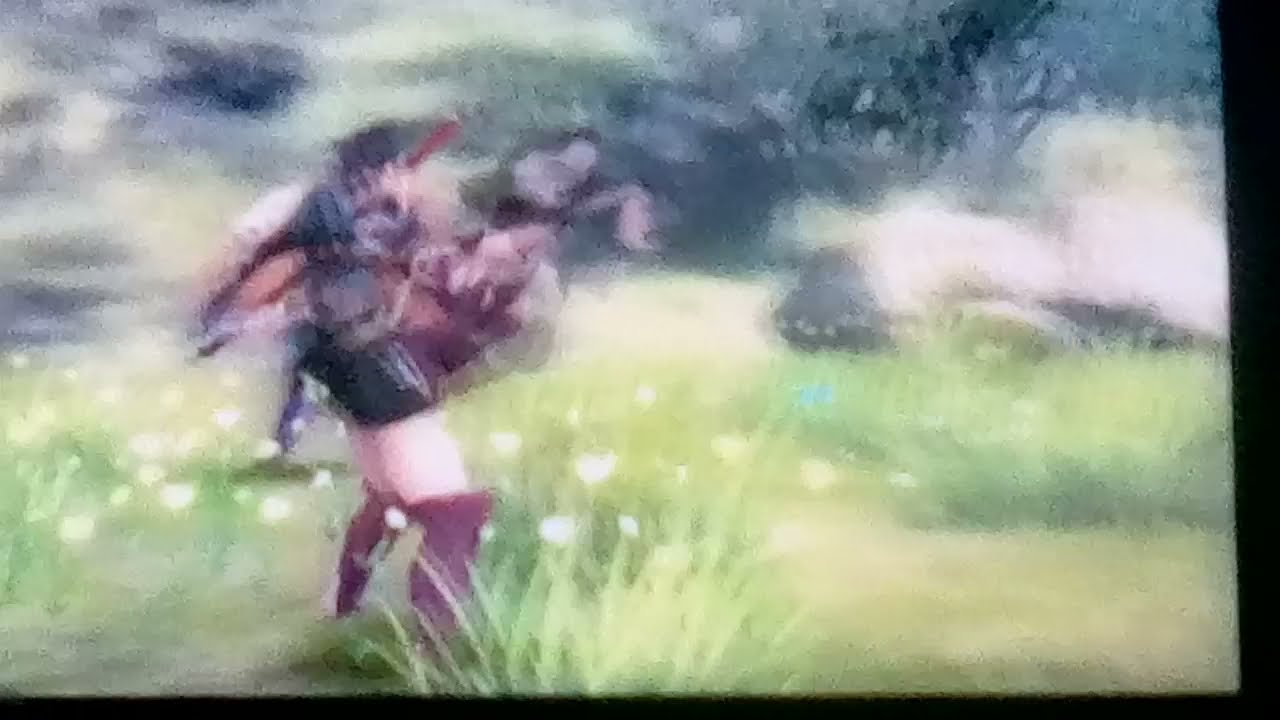This vertical rectangular image is very blurry, almost abstract, potentially capturing a scene from a photograph, a close-up of an impressionist painting, or even an image on a screen. The scene is set in a natural environment with tall green grass, dotted with white wildflowers. In the upper right corner, there appear to be large rocks or a fallen tree trunk, bathed in some sunlight with a backdrop of dark green trees and forestry. The left third of the image features a somewhat discernible figure, potentially a character with human legs wearing tall, knee-high red boots and short pants, and possibly adorned in dark red and purple attire. The figure's upper body is bird-like, or they might be carrying something, with a spiky short black haircut visible atop the head. The scene evokes a calm, almost video game-like ambiance, but the extreme blurriness makes the finer details very hard to make out, leaving much to interpretation.